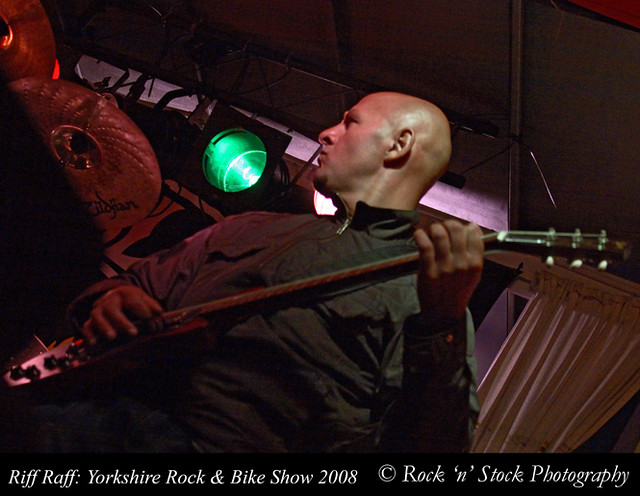This detailed photograph captures a bald musician on stage, clad in a black shirt with a zipper, playing an electric guitar while gazing slightly to his right. A green stage light is visible to the left of his face, casting a vivid illumination over the scene. Behind him, white curtains contrast sharply with the dark, possibly unfinished ceiling, where rafters are clearly exposed. In the background to his left, drum cymbals subtly hint at the presence of a drum set. The photo has been taken from an unusual angle, likely from a seated position, contributing to its unique perspective. Below the image, a black rectangular band features elegant white text that reads "Riff Raff; Yorkshire Rock and Bike Show 2008" followed by "Rock and Stock Photography," indicative of the event and the photographer.